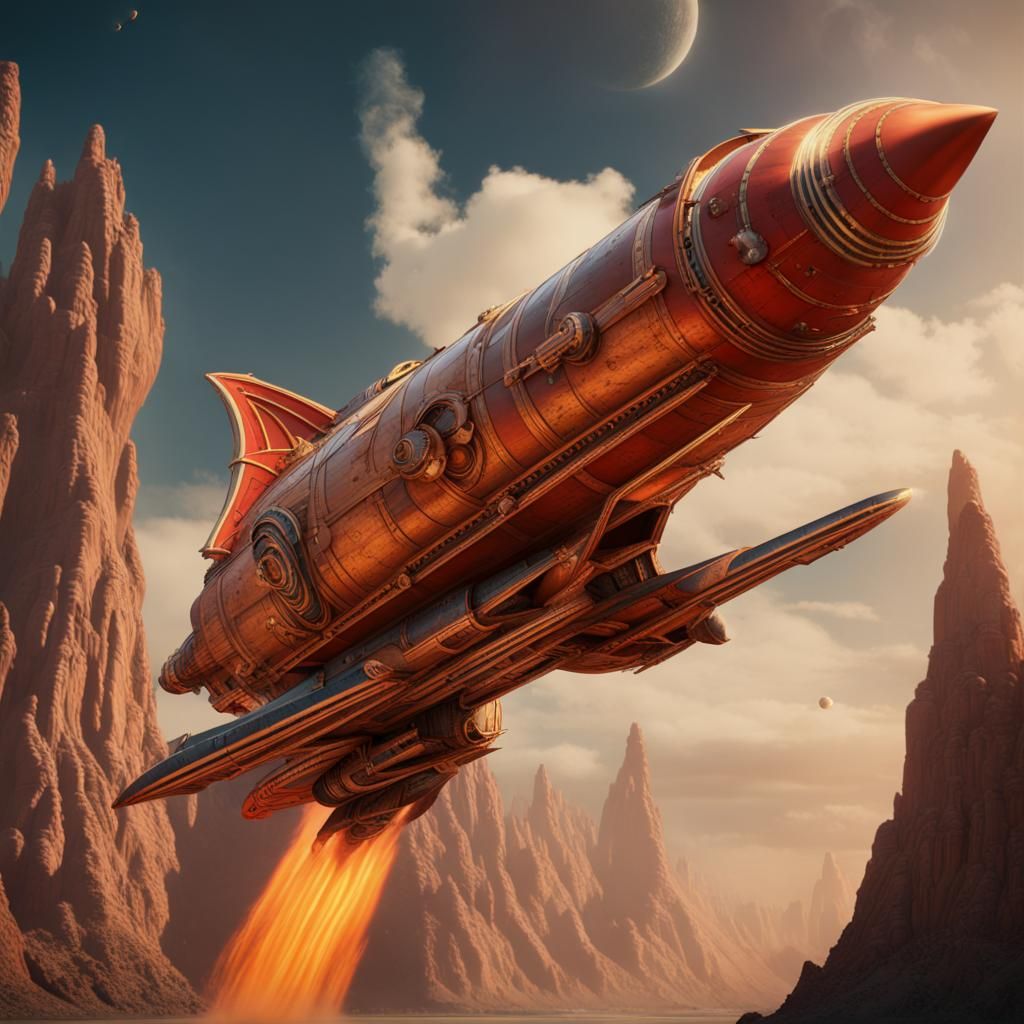The image features a large, elongated rocket ship with a shiny, copper-toned body, adorned with metallic rings around its length. The rocket's sharp, red-tipped nose contrasts with its overall copper and silver color. It features a unique fin at the top and dual steel-like wings at the bottom. Flames and orange light burst out from the rear, indicating its dynamic motion. The background showcases a rugged, arid landscape dominated by tall, pointy, brown mountain peaks that stretch diagonally from the bottom right to the top left. A smoky haze envelops the mountains, enhancing their jagged contours. Overhead, a dark blue sky is filled with thick, white clouds and a faint image of a white planet, completing the striking scene.